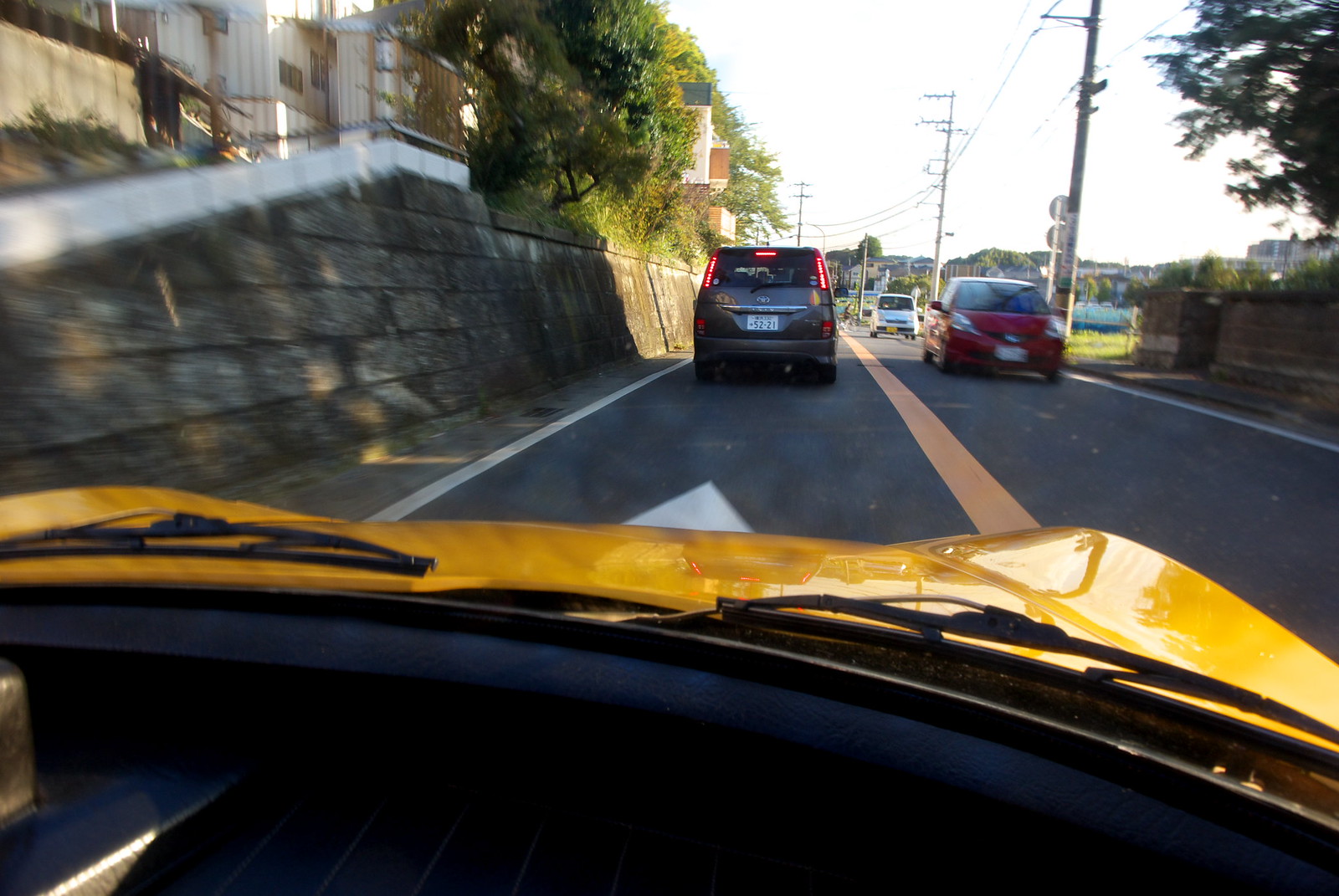A photograph, likely captured from a dashboard camera inside a moving vehicle, depicts a dynamic street scene. The left side of the image is notably blurry, enhancing the sense of motion, while the right side is moderately blurred, particularly the red car approaching the viewer's yellow car. The setting is on a gray road with a dual-lane layout, separated by a single, thick yellow line that traverses the entire road.

Directly ahead, a gray van with illuminated red brake lights can be seen. In the distance, the sun casts a golden hue on an array of vibrant green trees blanketing a nearby hill. Also approaching in the opposite lane, trailing the red car, is a white van.

Flanking the road, robust stone walls add a rustic charm, juxtaposing the lively traffic against a backdrop that quietly reflects the natural and constructed environment.